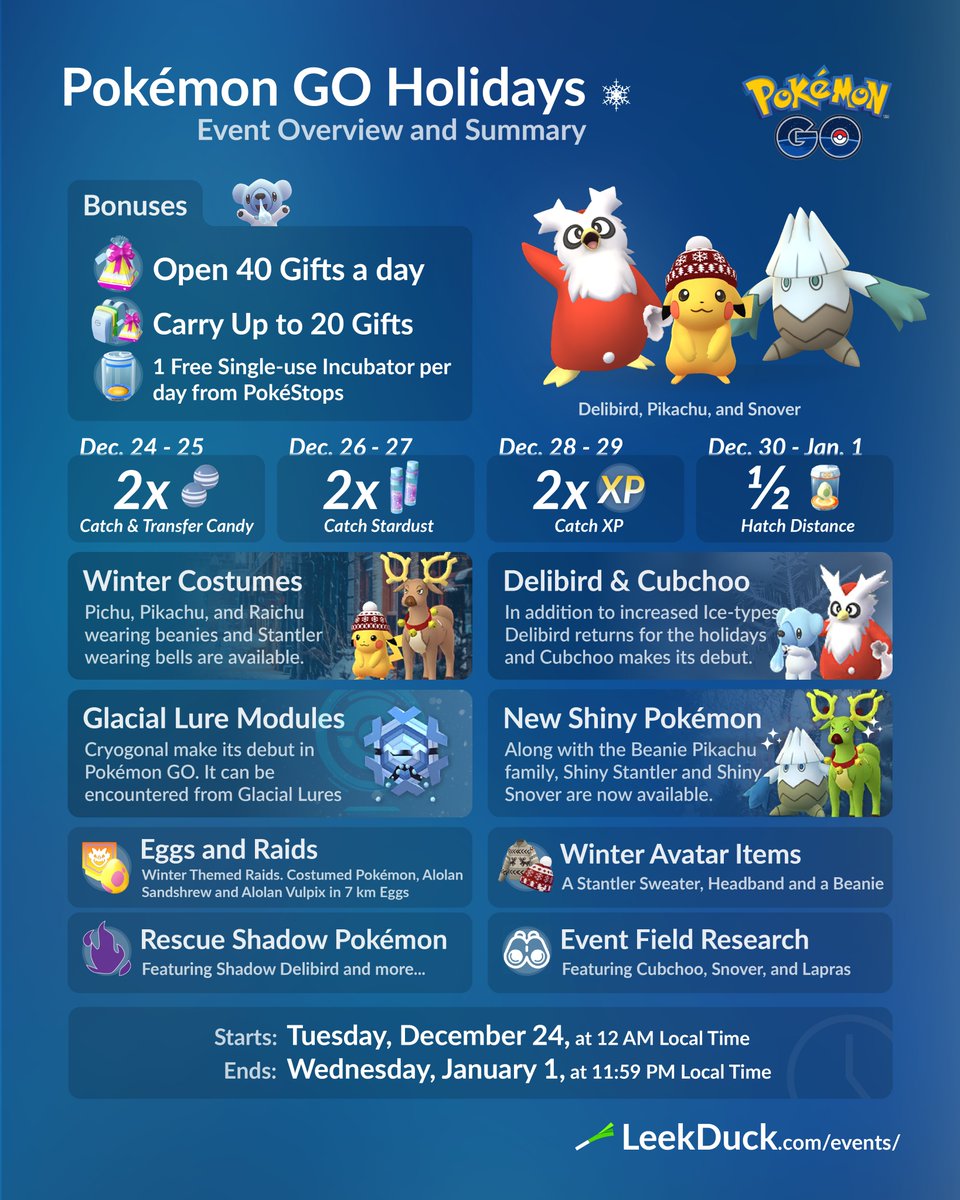The image features a predominantly blue background with white text detailing the Pokemon Go Holidays event. "Pokemon Go Holidays" is prominently displayed at the top along with "Event Overview and Summary" in yellow font on the right side. Featured characters include Delibird, Pikachu, and Snover. Delibird is depicted as orange and white, with wide eyes. Pikachu, recognizable by its yellow color and orange cheeks, is wearing a winter hat. Snover is egg-shaped with a gray, white, and teal color scheme.

The event offers numerous bonuses:
- Open up to 40 gifts a day.
- Carry up to 20 gifts and receive one single-use incubator per day from Pokestops.
- On December 24th and 25th, enjoy two times Catch and Transfer Candy.
- On December 26th and 27th, there's double Catch Stardust.
- From December 20th to 29th, players can earn double Catch XP.
- From December 30th to January 1st, benefit from half hatch distance for incubating eggs.

Additionally, the image showcases winter costumes including a reindeer outfit and a Pikachu in festive attire.